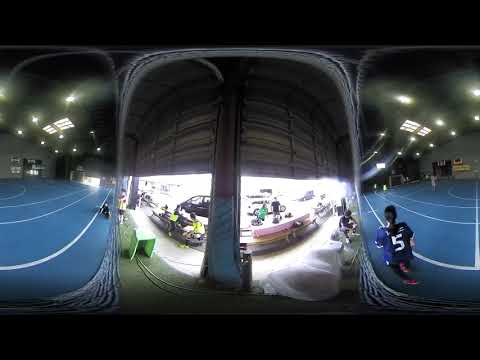The image is a small, almost square photograph taken with a lens that causes significant distortion, creating a somewhat disorienting effect. At the center of the image is an indoor track with a distinctive blue surface, bifurcated into lanes by white dividers. There is an individual in the lower right quadrant wearing a dark blue jersey emblazoned with the white number five, walking in the outer lane of the track. This person has dark hair.

On the left side of the image, a group of people is seated on a bench, apparently wearing fluorescent yellow safety jackets. Near them is a low green box table, adding to the scene's cluttered feel. A notable feature is a rolling garage door in the middle, which appears split, opening to a brightly sunlit exterior. Outside, the sunlight illuminates what looks like a car and some miscellaneous objects, possibly pallets, while a few people stand around.

Further adding to the complexity are the indoor lighting fixtures, or spotlight cans, affixed to the ceiling, casting light on the dim interior space. The distorted perspective of the image suggests it may have been taken with a 360-degree camera, capturing various elements like the dark indoor ceiling, the blue track, the open garage doors, and the bright outdoor scene, all within a confined frame.